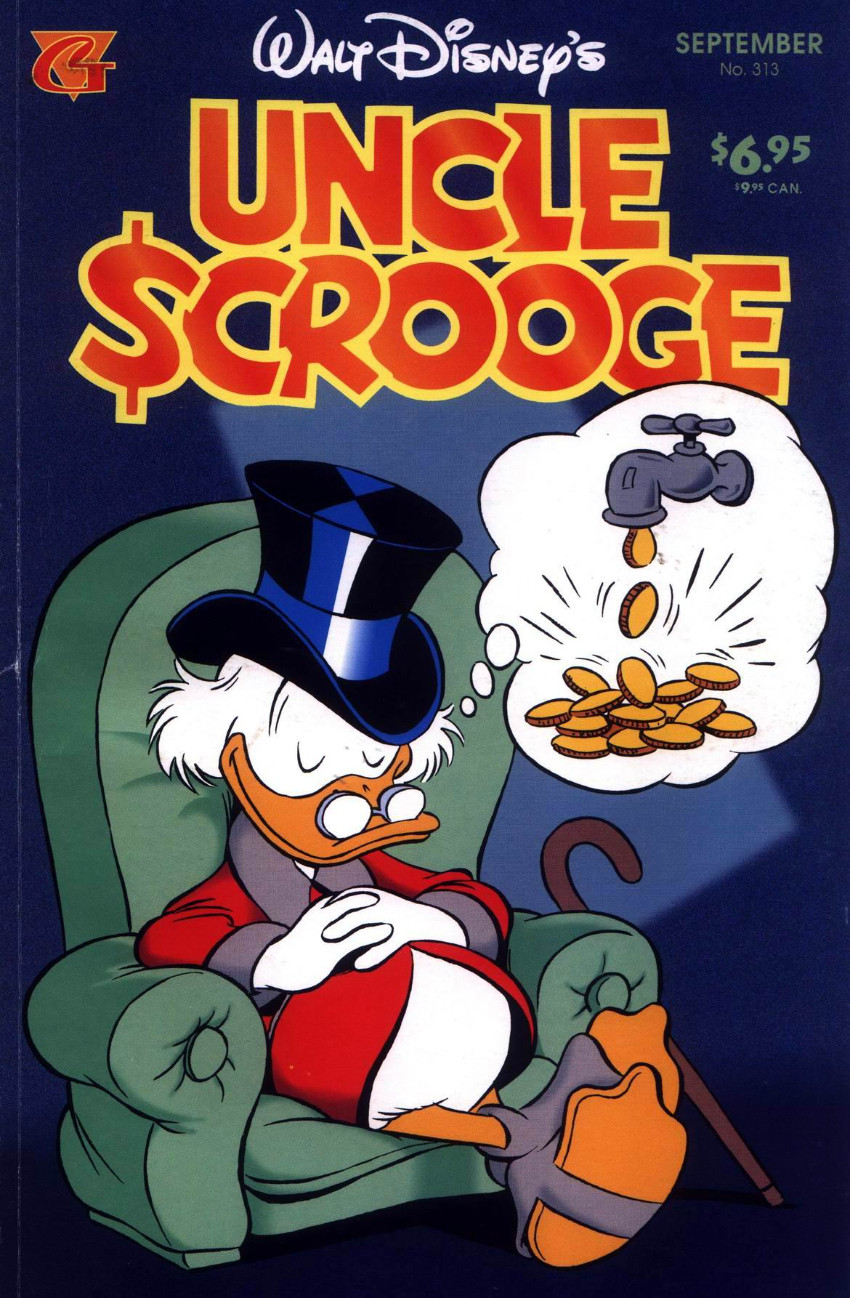The comic book cover features a DuckTales-themed design centered around the classic Disney character, Uncle Scrooge. Against a dark blue backdrop with a light blue rectangle angled diagonally, multiple text elements frame the scene. In the top left corner, a red triangle points downward with a large red letter "G" overlaying it. At the very top center, "Walt Disney's" is elegantly scripted in white cursive font. The top right corner announces "September, No. 313" in green printed font. Just below, in bold red text with a yellow border, the title "Uncle Scrooge" is prominently displayed, with the 'S' styled as a dollar sign. To the side, orange-green text indicates the prices "$6.95" and "$9.95 CAN."

Dominating the lower portion of the cover, Uncle Scrooge McDuck, clad in a red robe with purple accents and a black top hat, reclines in a green chair. His white feathers contrast with his orange bill and feet, giving him a distinguished appearance enhanced by the small glasses on his bill. Leaning against the chair is a brown cane, and above Scrooge's head, a thought bubble shows a dripping faucet pouring gold coins, symbolizing his endless wealth.